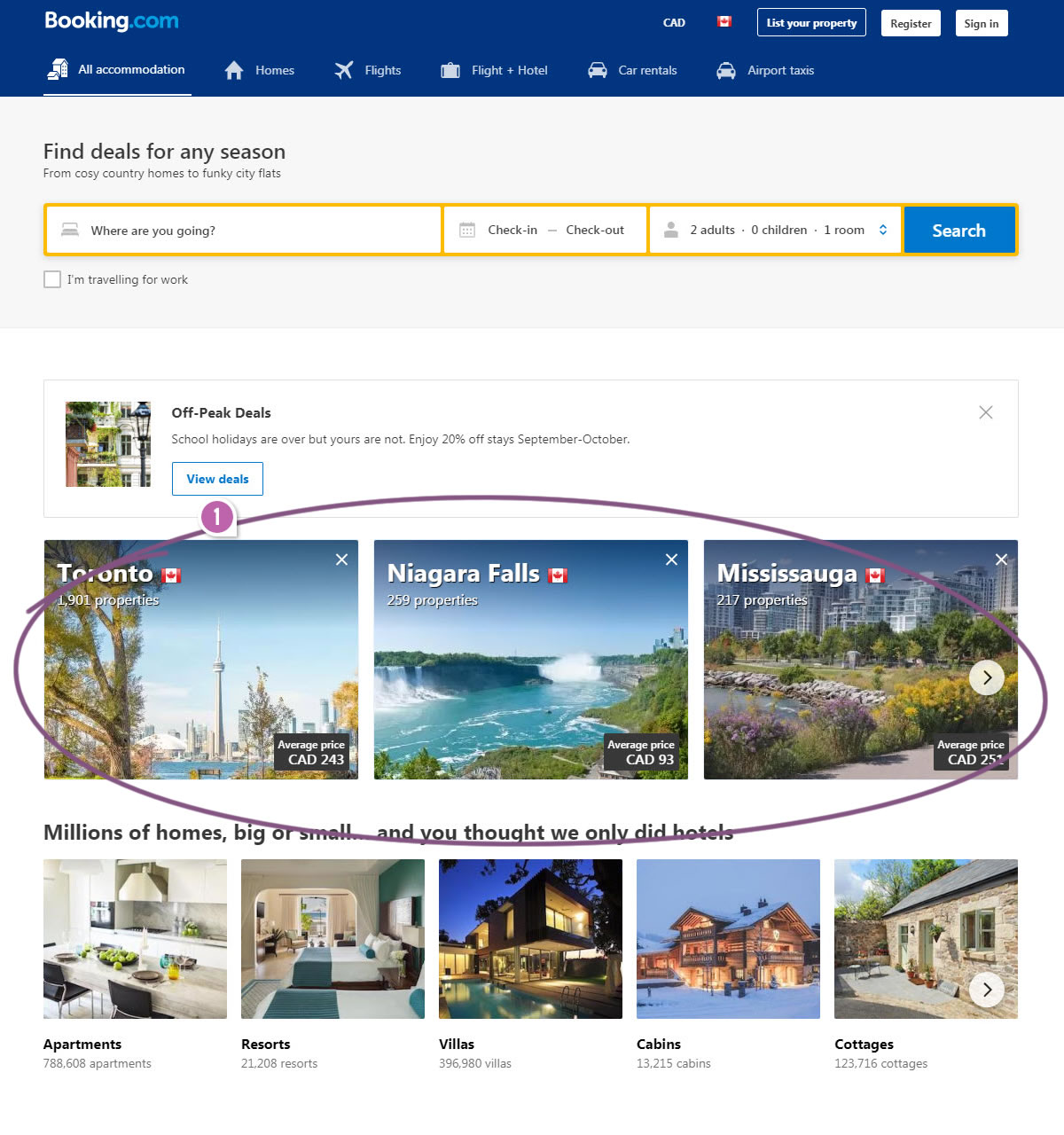The image is a screenshot of the homepage of the website Booking.com. At the top of the page, there is a prominent blue header featuring the Booking.com logo on the left side. Directly below this header, a navigation bar provides various options for making reservations, including "Stays," "Flights," "Flight + Hotel," "Car rentals," and "Airport taxis."

Underneath the navigation bar, a banner invites users to "Find deals for any season," highlighting the range of accommodations available—from cozy country homes to funky city flats. Below this banner, there are interactive boxes designed to help users customize their search. These include fields for entering a destination ("Where are you going?"), selecting check-in and check-out dates via a calendar tool, and specifying the number of travelers, including adults, children, and rooms. A prominent "Search" button enables users to initiate their search based on the entered criteria.

Further down the page, a section titled "Off-peak deals" offers suggestions for affordable travel periods. This section showcases a series of visually appealing destination options, complete with enticing images. Featured destinations include Toronto, Niagara Falls, and Mississauga.

Toward the bottom of the page, a message underscores the variety of lodging options available through Booking.com, stating, "Millions of homes, big or small, and you thought we only did hotels." The site highlights its diverse offerings, which include apartments, resorts, villas, cabins, and cottages.